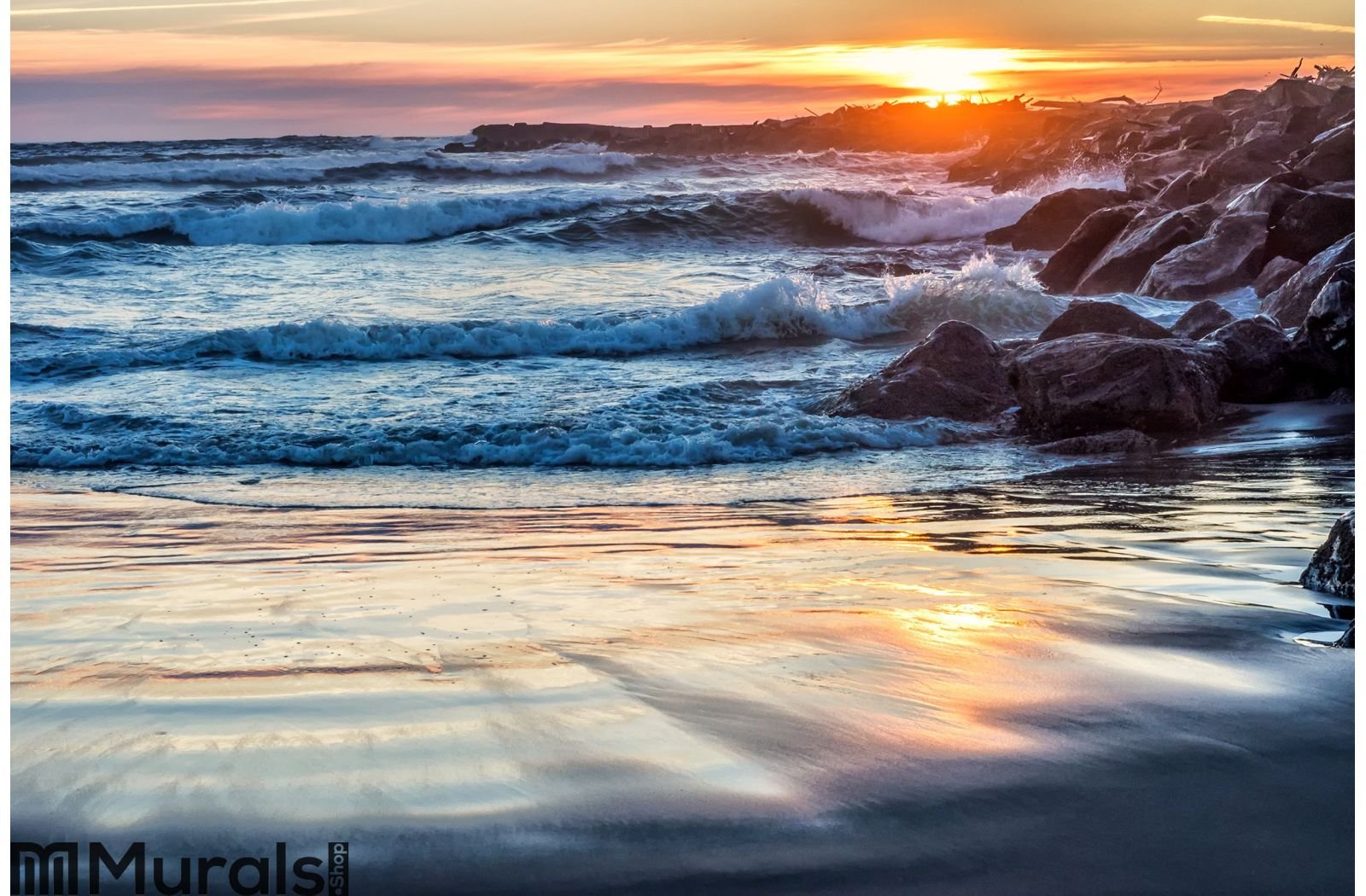This horizontally aligned rectangular photo captures a breathtaking beach scene during sunset. At the top of the image, the vibrant sky features a rich palette of brown, coral, gray, and pink hues. In the upper right section, a blob of yellow reveals the sun peeking out from behind the clouds. Below, on the left side, rough waves with white tips crash into the shore, their bluish-gray color contrasting against the dark expanse of water. Dominating the upper right side is a large formation of dark brown rocks extending toward the horizon. The entire bottom half of the picture showcases the wet, packed sand of the shoreline, mirroring the sun's reflection and creating a blend of brown tinged with light yellow. In the lower left corner, black print with a logo in the shape of an "M" and the word "MURALS" can be seen.